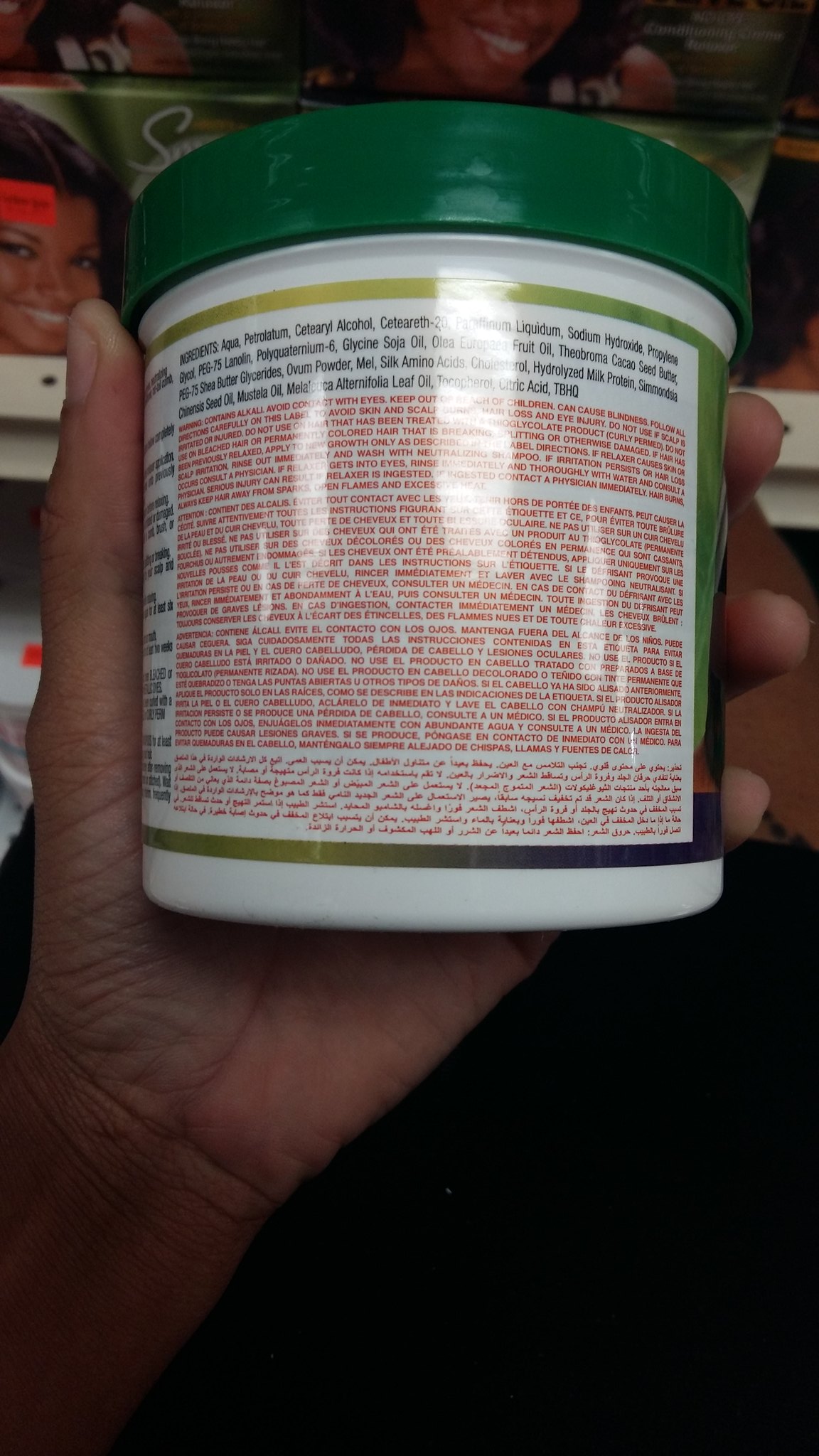A person is holding up a green plastic container with a green screw-on lid in their left hand. The container label, which they are showing, lists ingredients including aqua, petrolatum, cetearyl alcohol, and sodium hydroxide. Below the ingredients, there's a red warning label stating it contains alkali, advising to avoid eye contact, keep away from children, and follow directions to prevent skin, scalp, and hair damage. The warning is also translated into multiple languages. The person is taking the portrait-style photo with their right hand in what appears to be a store, as shelves with various products and visible price tags are in the background, suggesting it might be a beauty shop.